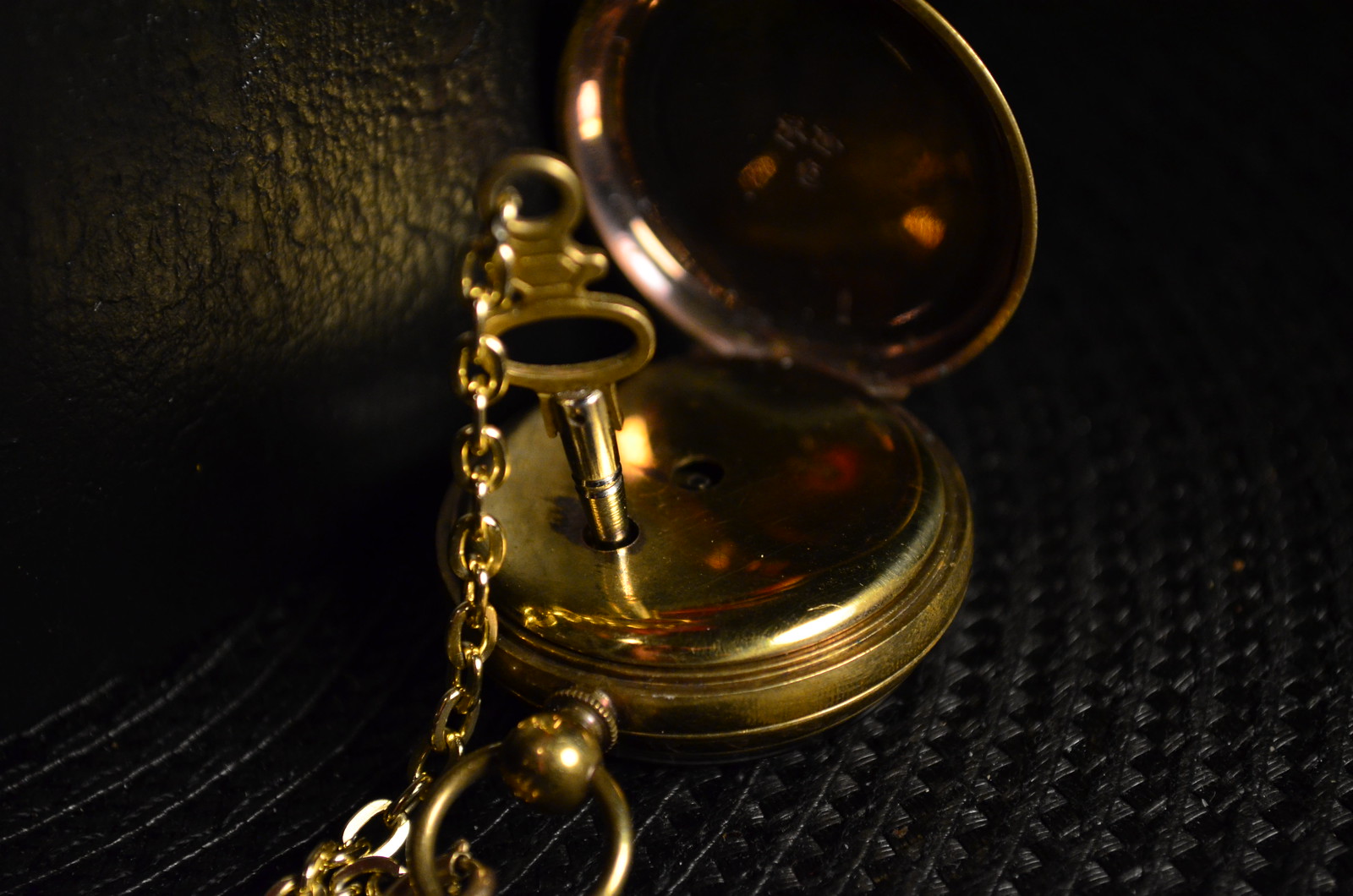The image captures a close-up, artistic photograph of a vintage pocket watch, predominantly gold or brass in color, laid open on a dark, almost black surface with a striped, ribbed pattern. The pocket watch, small and circular in shape, features an intricately designed gold plate inside, with no visible numbers. A key is inserted into a slot on the watch to wind the mechanism, suggesting the watch is in need of winding. This key is connected to a long gold chain, typically used to hang the watch from a pocket, and is likely removable. The surface beneath the watch appears to be composed of fibrous woven material with concentric rings, adding texture to the image. Adjacent to the pocket watch is a wall with a greyish-gold hue, providing a complementary backdrop to the scene. The overall composition emphasizes the intricate details and craftsmanship of the timepiece, set against contrasting textures and tones.